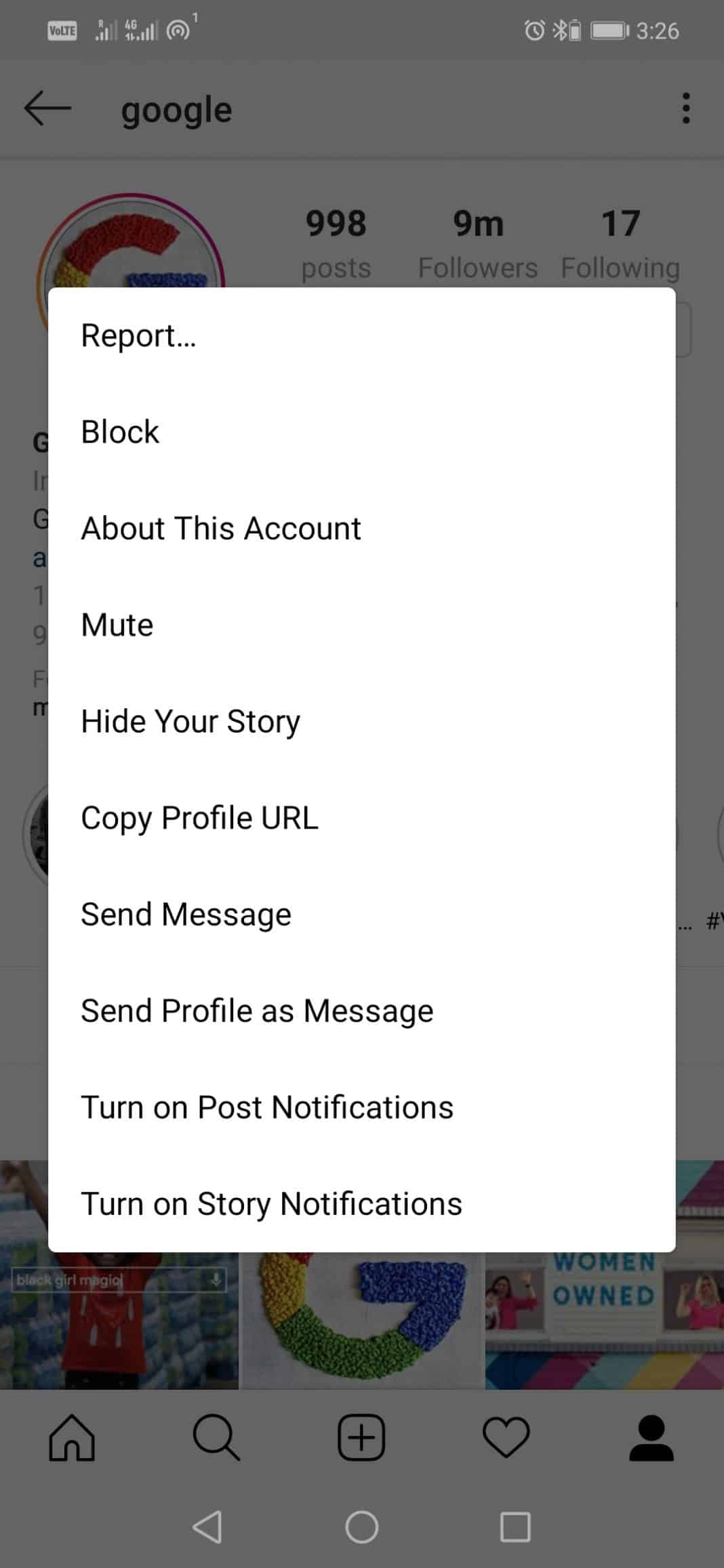The image displays a smartphone screen, presumably within the Google app. At the top of the screen, the time is shown as 3:26, accompanied by various notification icons, including Bluetooth, an alarm clock, and other unidentified symbols.

Just beneath the notification bar, the Google logo is prominently displayed in lowercase letters paired with the colorful 'G' symbol. The profile metrics are listed below it, indicating 998 posts, 9 million followers, and 17 following. 

Above the profile metrics, there is a pop-up menu providing options such as "Report," "Block," "About this account," "Mute," "Hide your story," "Copy profile URL," "Send a message," "Send profile as message," "Turn on post notifications," and "Turn on story notifications."

Below this section, in a clear white box, is the tag "Women Owned," the Google 'G', and possibly a small photograph of a person. At the very bottom of the screen, there is a navigation bar featuring icons for "Home," "Search," "Add (plus sign)," "Heart," and "Profile (a small person symbol)."